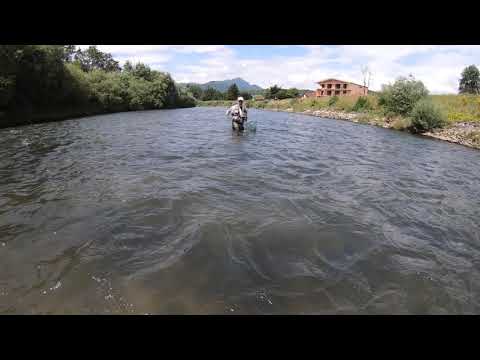In this out-of-focus landscape photo, a fly fisherman stands mid-stream in a gray, rippling waterway. Clad in waders, a white hat, and a white long-sleeved shirt over black pants, the fisherman holds a fishing pole and has one hand raised near his chin. On the right bank, there is a pink, two-story building resembling a lodge or cabin with an arched roof. The scene is framed by dense vegetation: thick, green-leaved trees dominate the left side, and lighter green grass along with a couple of darker shrubs and a tall tree are seen on the right. In the distance, we can see blue-hued mountains under a partly cloudy sky with white clouds. The photo is landscape-oriented, capturing the serene natural setting under midday light.